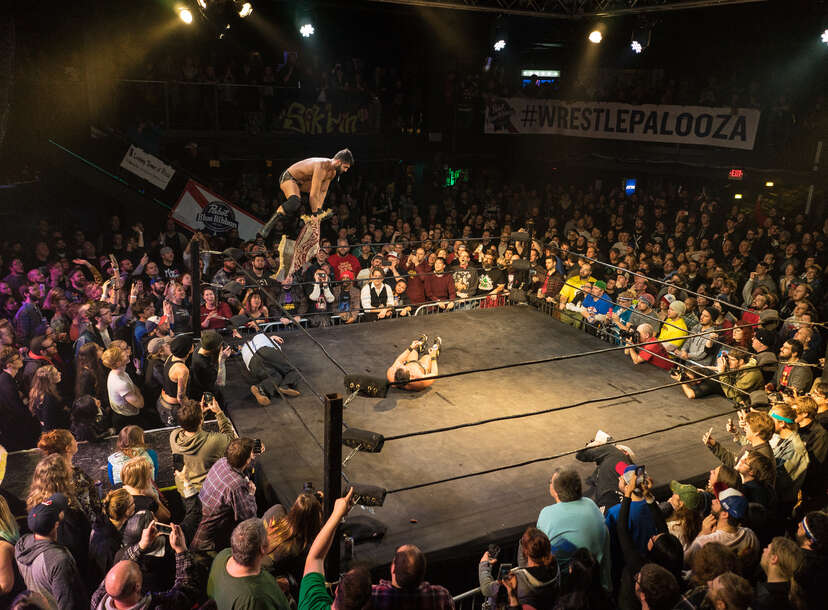This indoor photograph captures a dynamic moment at an event presumed to be "Wrestle Palooza," evident from a prominently displayed banner reading "#WrestlePalooza" held up by numerous spectators. The camera angle is from a higher vantage point, providing a comprehensive view of the wrestling ring and the surrounding audience. Within the ring, a dramatic scene unfolds as one man dives off the edge, poised to execute a maneuver on a prone opponent lying on the mat. The match's intensity is underscored by the presence of a motionless referee also on the mat, suggesting he may have been inadvertently knocked out. The audience encircles the ring, with spectators of diverse backgrounds filling the space, many intently watching the action without the distraction of phones, hinting it might be an older image. On the wall in the background, a “Blue Ribbon” sign, likely referring to a beer brand, adds a touch of nostalgia. Additionally, another shorter banner with yellow lettering can be seen, though its message is less clear. This image vividly portrays the excitement and chaos inherent to wrestling events, highlighting the passionate crowd and the high-stakes drama within the ring.